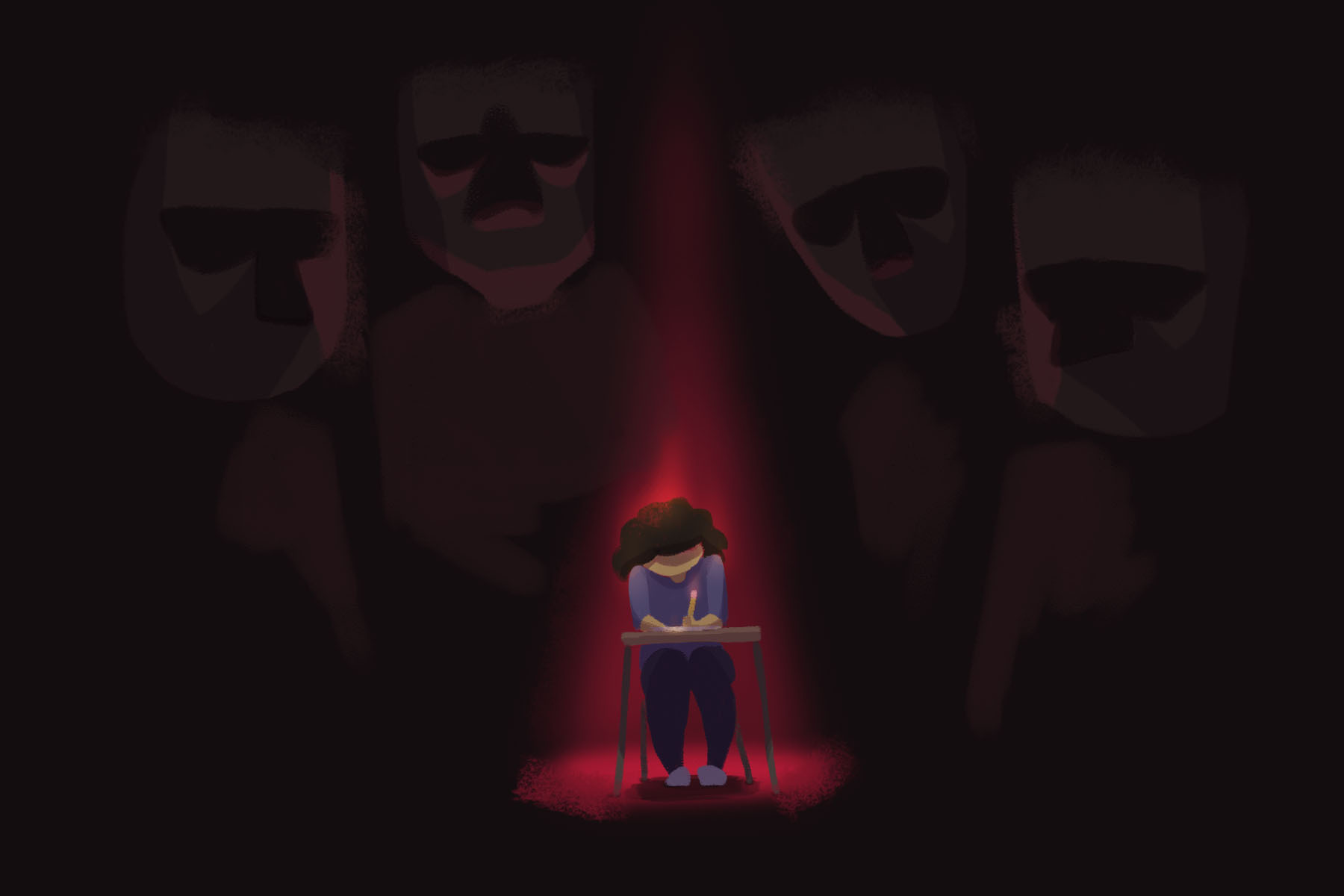In this dark and ominous cartoon-style image, a tan-skinned girl with black wavy hair is seated at a brown desk with dark brown legs, writing intently with a yellow pencil that has a pink eraser. She is adorned in a purple shirt, black pants, and lavender slippers. The scene is illuminated by a red spotlight that casts an eerie glow around her, emphasizing the sense of isolation on what appears to be a stage with a red floor. 

Above her hover four sinister masks, two on each side, bearing expressions reminiscent of the traditional comedy and tragedy theatrical masks. These masks gaze down at her as she concentrates on her writing, adding to the overall grim atmosphere. The backdrop is enveloped in complete darkness, further enhancing the feeling of unease and scrutiny as the girl works under the watchful eyes of the malevolent masks.